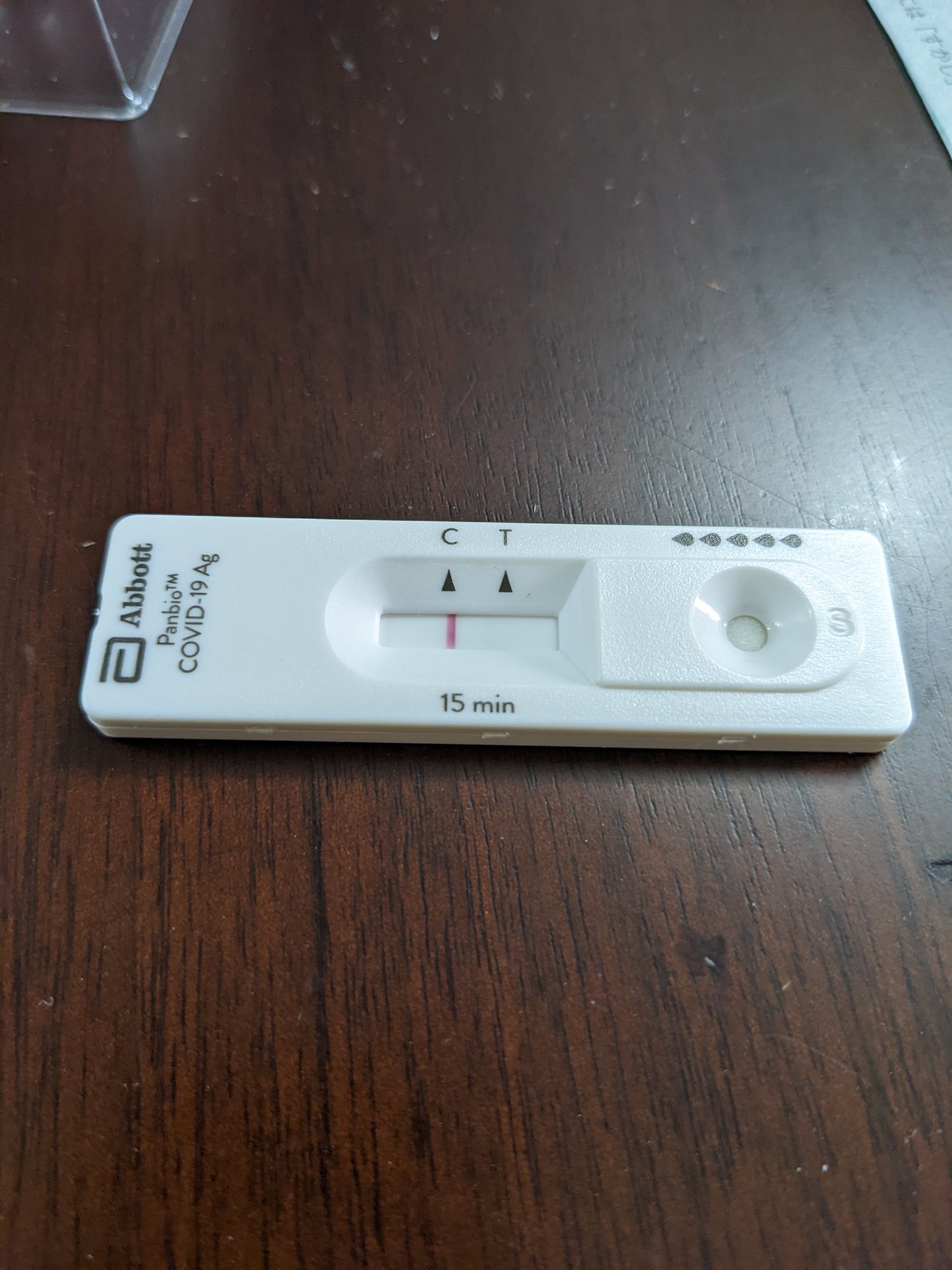The image features a Covid-19 test kit placed on a dark brown, finely grained wooden table that has darker brown and black stripes running through it. The table shows signs of use with noticeable stains toward its top, possibly from a spill. The Covid-19 test kit, oriented sideways, is predominantly white and labeled with “Abbott PanBio Covid-19 AG” at the top. 

Below the label, there is a small window with 'C' and 'T' markers flanking it; a single red line appears next to the 'C', suggesting a negative test result. An area designated for the application of test droplets is marked with small water droplets and is located near a small indentation at the bottom of the test kit. Three perforations are visible along its bottom edge. 

Also included in the frame, positioned in the upper right-hand corner of the table, is a small, square glass object. The Abbott logo, featuring a stylized black line resembling a backwards 'G', is placed adjacent to the brand name at the top of the test. The Covid-19 test kit is the central focus and the only item prominently displayed on the table.